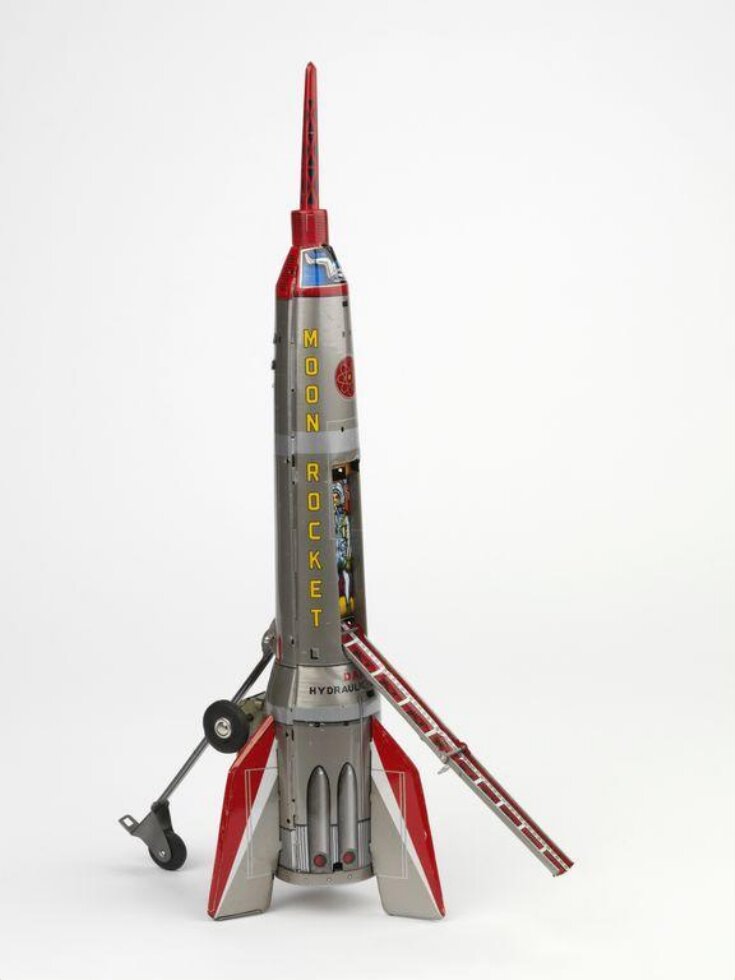This image features a color photograph of a vintage model rocket, likely from the early 1960s, set against a light gray background. The rocket itself is tall and predominantly metallic silver-gray, with a distinctly pointy, narrow nose painted bright red. Its body displays the text "Moon Rocket" in vertical yellow letters. Notably, the rocket includes three tail fins that are accented with red, white, and gray stripes. A red and white stairway or ladder extends from the rocket, implying access to an interior compartment. Visible through a small opening, there's a model astronaut complete with a helmet, suggesting a manned mission. The rocket also features wheels on one side, presumably for easy transport.